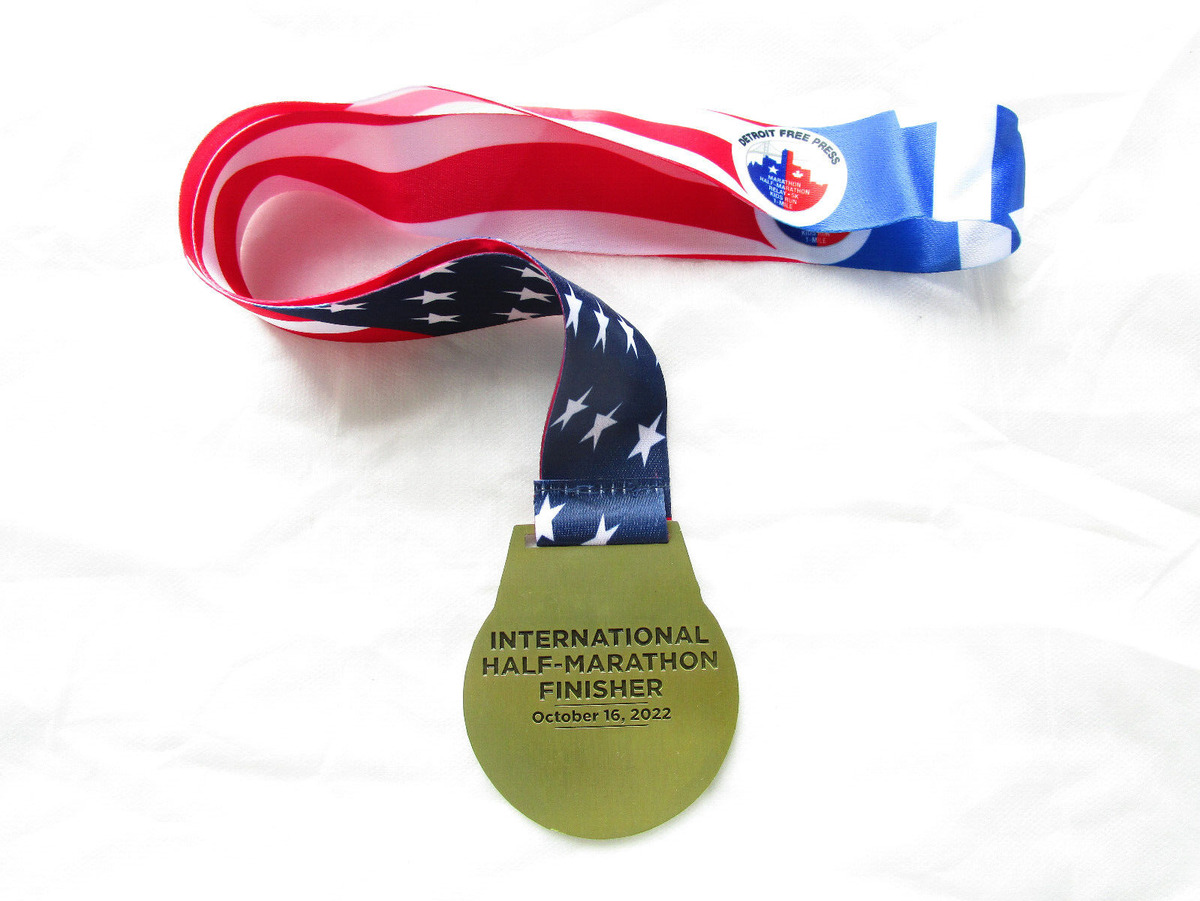This vertical image showcases a medal awarded for completing an International Half Marathon. The medal, which is gold-colored, is inscribed with the words “International Half Marathon Finisher” and dated October 16th, 2022. This medal is attached to a ribbon designed to resemble the American flag. The top portion of the ribbon, which forms a loop, is adorned with blue and white stars, while the rest of the ribbon features red and white stripes running up toward the neck area. Near the top of the ribbon, there is a sticker that reads "Detroit Free Press" along with an outline of skyscrapers split between blue and red colors, though some of the smaller text on it is not discernible. The medal and ribbon are folded in a T-shape against a plain white background, emphasizing the medal's prominence and the intricate design of the ribbon with its patriotic theme.